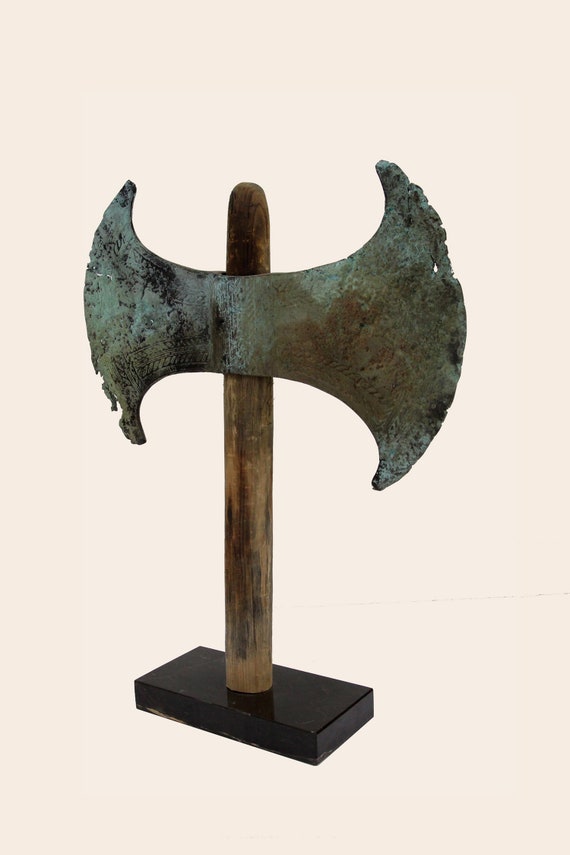This photograph captures a striking found object that has been artistically mounted to evoke the appearance of a sculpture. The centerpiece of the image is a large, double-edged axe with a wooden handle. The axe is positioned vertically on a modern black stone pedestal and appears to be placed indoors against a beige background, which may have a subtle pink or light brown tint. 

The axe itself has a weathered appearance; its blades exhibit noticeable rust and gouges, with hues of bluish-gray, rusted green, and brown, enhancing its ancient, almost archaeological, feel. The edges of the blades are worn and imperfect, with some areas showing chips and signs of crumbling. These details make the material difficult to pinpoint, as it could be metal or stone. The wooden handle, medium brown in color, shows stains and wear that add to the aged aesthetic. 

Overall, the image portrays an evocative blend of historical artifact and contemporary artistic presentation, providing a compelling visual narrative.